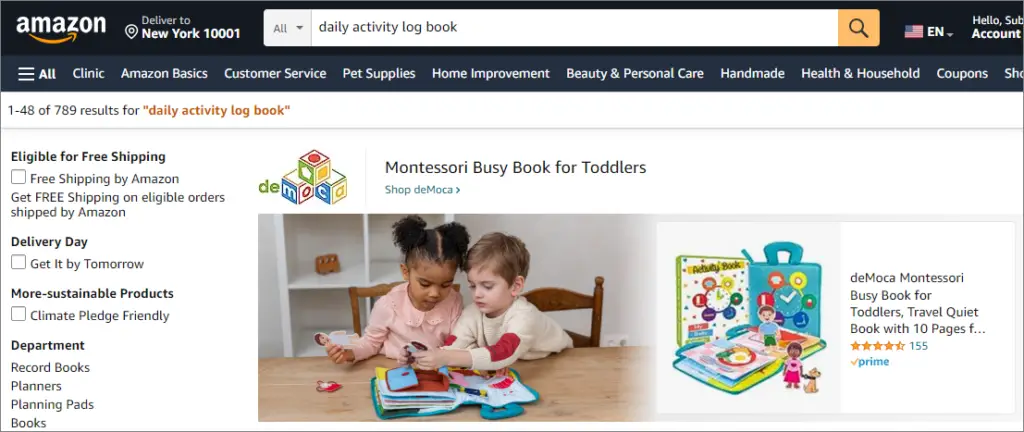This image is a screenshot from the Amazon website. At the top of the page, the background is black, featuring the white Amazon logo in the top left corner. Next to the logo, there is text stating "Delivered to New York 10001." The central part of the header includes a white search bar where the user has searched for "daily activity logbook." Adjacent to the search bar, there is an icon of a flag with "EN" displayed beside it, indicating the language setting. Further to the right, it reads "Hello, Account," suggesting the option to access the user's account details.

Below this header, there is a navigation menu offering various categories such as "All Clinics," "Amazon Basics," "Customer Service," "Pet Supplies," "Home Improvement," "Beauty & Personal Care," "Handmade," "Health & Household," and "Coupons."

Underneath this menu, a section states "1-48 of 789 results for daily activity logbook." Featured prominently in the middle of the page is a product listing for a "Montessori Busy Book for Toddlers." The listing includes an image of two young children engaging with the Montessori book, alongside a close-up image of the book itself, highlighting its design and details.